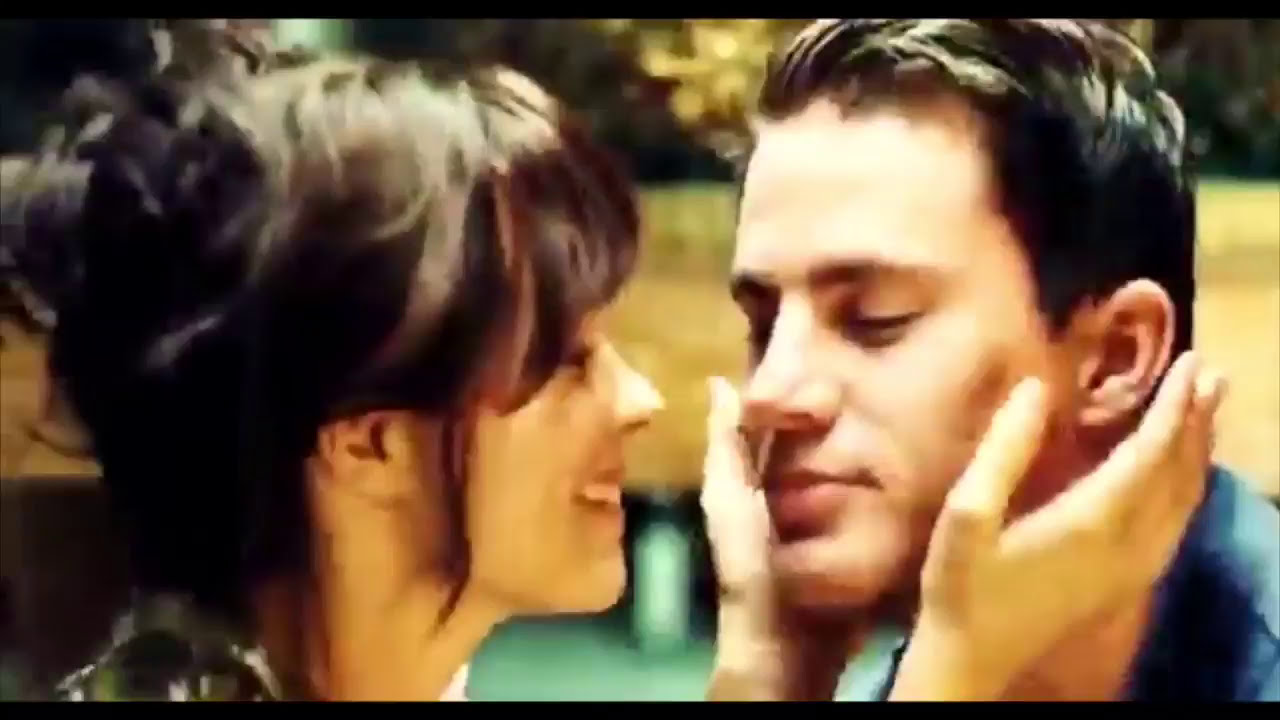A young woman, with dark brown hair tied up in a messy bun, stands on the left, facing a man on the right. She is gently cupping the man's cheeks with both hands, her face radiating warmth with a slight smile that reveals her teeth. The man, who bears a striking resemblance to Channing Tatum, has short black hair and his eyes closed, enjoying the intimate moment with a subtle smile playing on his lips. He is dressed in a blue polo shirt or t-shirt. The background features horizontal wooden boards with some trees visible above them, suggesting they are outdoors, possibly lit by daylight or studio lighting that creates minimal shadows and peculiar highlights. There is a sense of serene connection between them, making the scene feel like a tender still from a romantic movie.